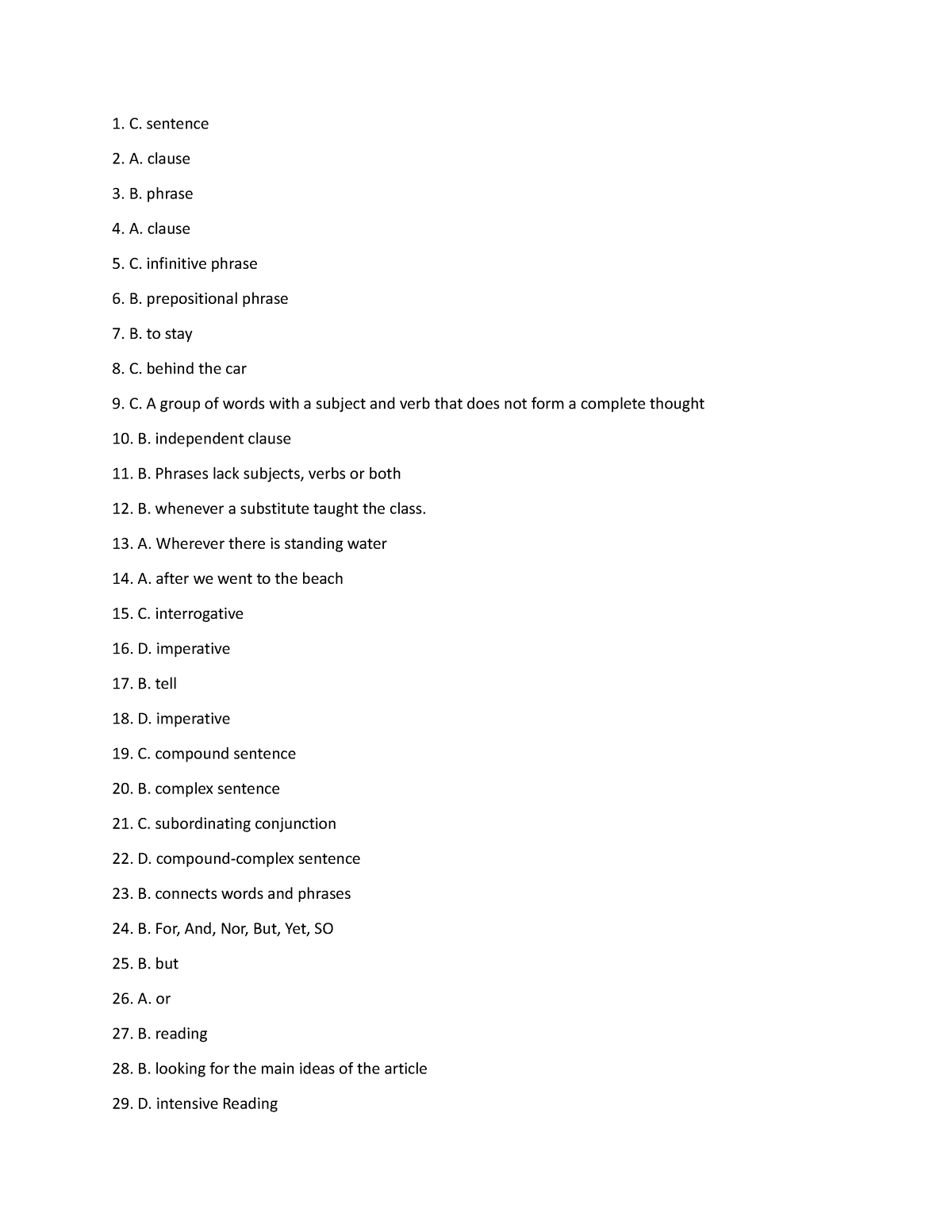The image depicts a neatly arranged list, numbered from one to twenty-nine, with each item written in black text. The list is divided into different sections, each beginning with a phrase and followed by relevant grammatical terms and examples.

1. At the top, a single "C" denotes a sentence.
2. Next, "A" indicates a capital phrase or clause.
3. "B" identifies a capital phrase.
4. The pattern continues, with "A" indicating another clause.
5. "C" describes an infinitive phrase.
6. "B" mentions a prepositional phrase.
7. The phrase "to stay" is labeled "B."
8. "Behind the car" is described as a prepositional phrase under "C."
9. A capital "C" introduces "a group of words with a subject and verb that does not form a complete thought."
10. "Independent clause" is marked as "B."
11. Under "B," it notes that "phrases lack subject, verb, or both."
12. "Whenever a substitute taught the class" is listed as "B."
13. "Whenever there is standing water" is an example of a clause under "A."
14. "After we went to the beach" is another clause, also under "A."
15. An "interrogative" sentence is denoted by "C."
16. An "imperative" sentence is marked as "D."
17. "Tell" is simply marked as "B."
18. Another "imperative" is noted as "D."
19. "Compound sentence" is labeled "C."
20. "Complex sentences" is marked as "B."
21. "Coordinating conjunction" is under "C."
22. "Compound complex sentences" are indicated with "D."
23. Finally, "B" stands alone without additional context at item number twenty-three.

This meticulous enumeration, with its emphasis on grammatical structures and varied sentence types, likely serves as an instructional reference for language learning or linguistic analysis.